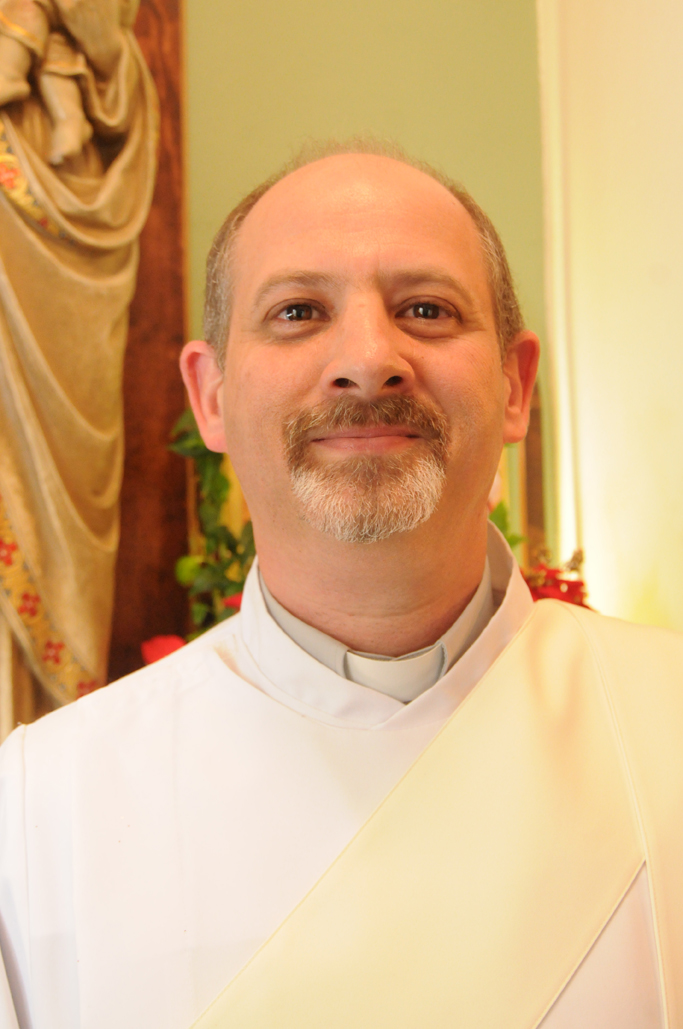The image depicts a middle-aged man of Caucasian or possibly Middle Eastern descent with a light complexion. He is standing in a church environment, posing for a close-up photograph. The man is smiling warmly at the camera, which is angled slightly upwards from a straight-on perspective. He has dark brown eyes, is balding at the front, and has light brown hair with white strands interspersed both on his head and in his goatee, which includes a mustache and facial hair on his chin.

He is dressed in religious attire, indicative of someone in training or service within the church, such as a vicar or priest. The man is wearing a light gray shirt with a plastic priest collar, over which he has a white robe. He also has a yellowish-cream or beige sash draped over his left shoulder, crossing his torso. Behind him, the background suggests a chapel setting, with a pale-colored statue resembling the Virgin Mary holding baby Jesus. A curtain and part of a wall are also visible to the left of the man in the background. The photograph seems to be taken possibly as part of a ceremony or for a publication highlighting his role within the church.